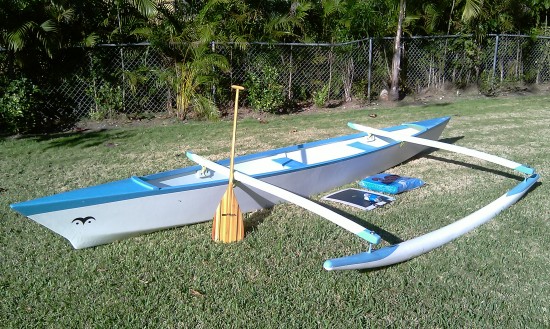In the image, there is a prominent, long-looking canoe, intricately detailed with a white bottom and a sky blue trim on top. The canoe is equipped with two slender rods protruding from the side, possibly serving as stabilizers. Alongside the canoe, there is a beautiful, light-colored wooden paddle propped up against it, standing upright. Also near the canoe, there seem to be seat cushions lying on the grass, suggesting additional accessories for use with the canoe.

The setting is a grassy area with a mixture of vibrant green and patches of dry, brown grass, indicating some wear. In the background, a metal chain-link fence is visible, standing in front of a lush, green treeline, adding a natural, forested backdrop to the scene. The bright white and blue colors of the canoe stand out vividly against this verdant and slightly rugged environment, making it a striking focal point of the image.